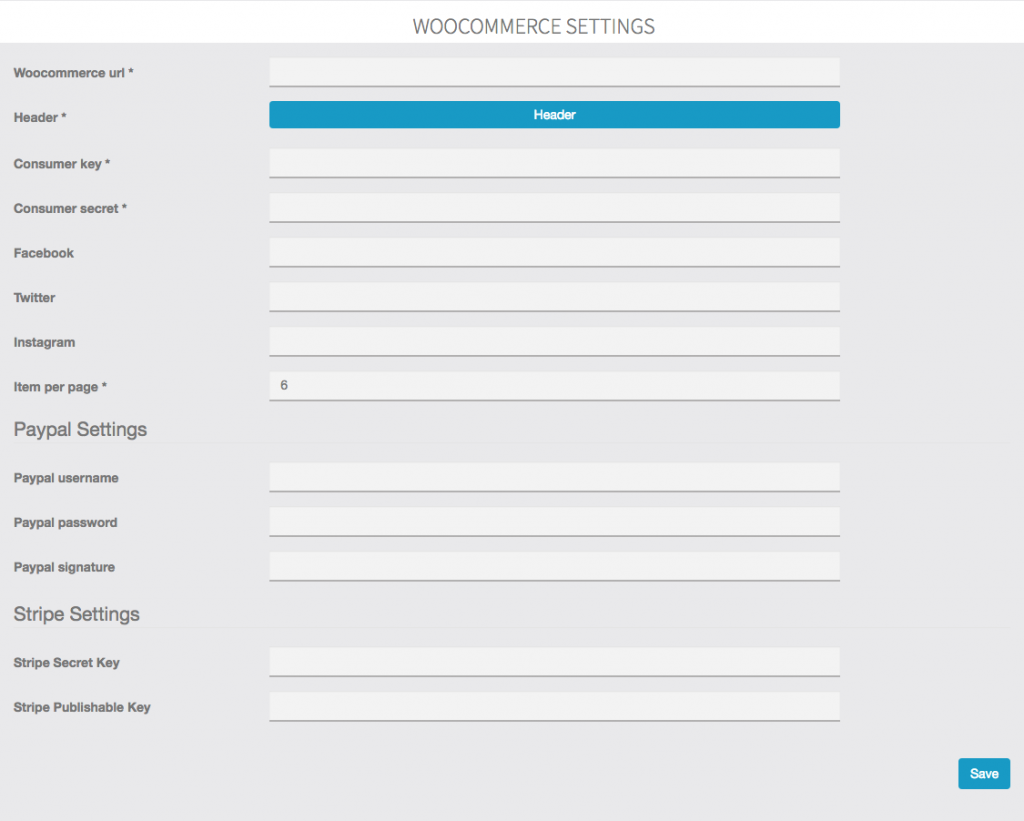This image showcases the settings page for WooCommerce, an e-commerce plugin for WordPress. The page features a gray background with multiple input fields organized in a list. The input labels are displayed on the left side in gray text. The second item on the list deviates from the standard format by displaying a blue button labeled "Header" instead of a typical input field. 

The list of input labels includes:
- WooCommerce URL
- Header
- Consumer Key
- Consumer Secret
- Facebook
- Twitter
- Instagram
- Items Per Page
- PayPal Settings
  - PayPal Username
- Stripe Settings
  - Stripe Secret Key

At the bottom right corner of the page, there is a prominent blue button with white text that reads "Save." This button likely serves as a means to apply any changes made on this settings page.